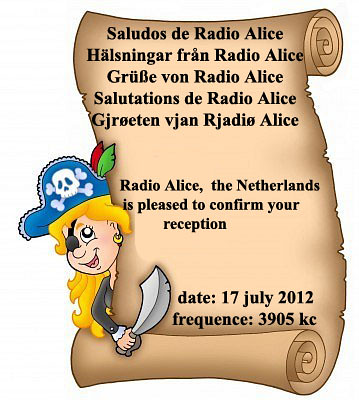This image presents an artistic digital illustration featuring a parchment scroll and a female pirate avatar. The parchment, rendered in shades of brown with curled edges—curled behind at the top and in front at the bottom—is centered in the composition. It bears black text, with a header in a non-English language, followed by the message: "Radio Alice, the Netherlands is pleased to confirm your reception. Date: 17 July 2012, Frequency: 3905 KC."

Peeking from behind the left side of the scroll is the digital avatar of a smiling pirate girl. She is characterized by her vibrant blonde hair, peach skin, and a striking blue pirate hat adorned with a white skull and crossbones, along with two feathers—one green and one red. She wears a black eyepatch over her right eye and a gold earring in her left ear. Dressed in a black shirt with white linen accents, she holds a sword with a dark and light gray blade in her right hand, positioned prominently above the scroll. This playful and detailed depiction stylizes the presentation of the message as if transmitted through a whimsical, pirate-themed digital artwork.